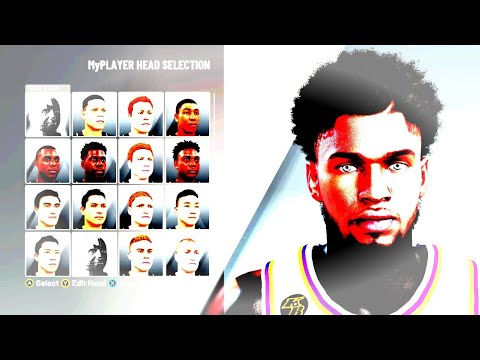The image appears to be a screenshot from a video game, specifically a character selection screen. The scene is framed by thin black bars at the top and bottom, providing a cinematic effect, and is set against a white background. 

In the upper left-hand corner, there is a light gray outlined box labeled **"My Player Head Selection"** in white text. This box contains four rows, each with four headshots, offering a total of sixteen character choices for customization.

- **First Row**:
  1. Black and white photograph
  2. Man with short black hair
  3. Red-headed man
  4. African-American man with short hair

- **Second Row**:
  1. Black man with short hair
  2. Black man with slightly longer black hair
  3. White man with red hair
  4. Black man with slightly longer black hair

- **Third Row**:
  1. Caucasian man with short dark hair
  2. Man with yellowish skin tone and long black hair in a ponytail
  3. White man with red hair
  4. Asian man with short dark hair

- **Fourth Row**:
  1. Asian man with short hair
  2. Oversaturated black and white photo, where the face is barely visible
  3. Caucasian man with red hair
  4. Caucasian man with a buzz cut

Below the head selection box, there are options for **"SELECT"** and **"EDIT HEAD,"** marked by a yellow and green circle, respectively.

On the right-hand side is a larger, highlighted image of the selected character. This character is an African-American man with slightly longer black hair—neither buzz cut nor long. He sports a thin mustache, blue eyes, and a black beard on his chin. His neck, which appears darker than his face, hints at possible neck tattoos. He is dressed in a white basketball jersey featuring purple and yellow stripes along the neck and shoulders, following a tank top style.